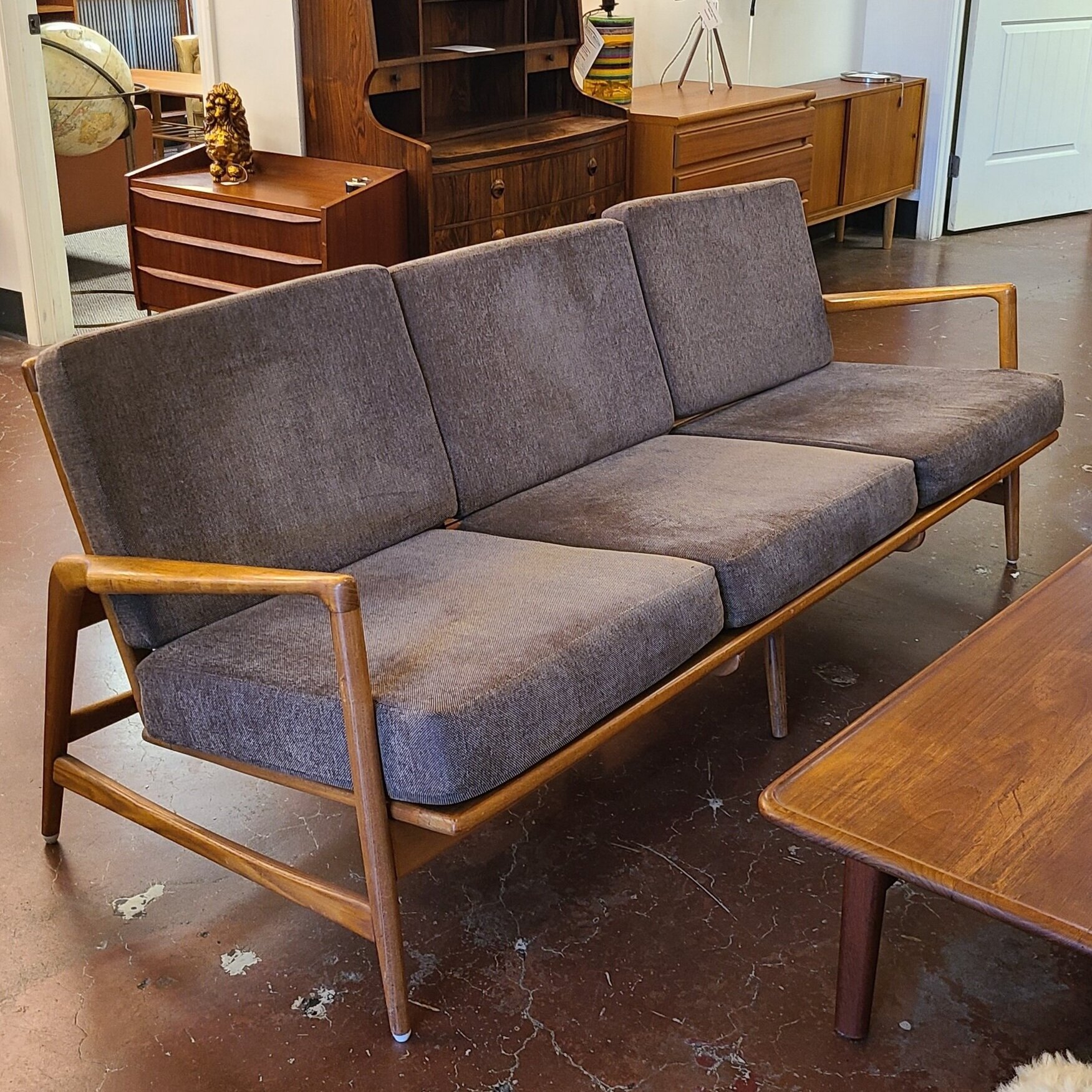In the photograph, a focal point is a simple gray futon with three rectangular, neatly positioned, velour-like cushions, framed by semi-polished wooden arms and legs. The structure evokes a mid-century modern design. Positioned on a worn, chipped concrete floor, the futon is complemented by a matching wooden coffee table set immediately in front.

The background reveals an assortment of furniture, possibly from a sale or estate event, as several pieces bear indistinguishable tags. Close behind the futon, we see several credenzas and cabinets, cluttered together and topped with knickknacks, including a golden poodle statue, a bust, a carving, a lamp, and a round silver dish. In an adjacent room visible through an open doorway, an old globe with yellowed oceans adds a vintage touch to the scene. Further adding to the eclectic array are additional wooden desks and tables, reinforcing the suggestion of a furniture sale or estate liquidation.